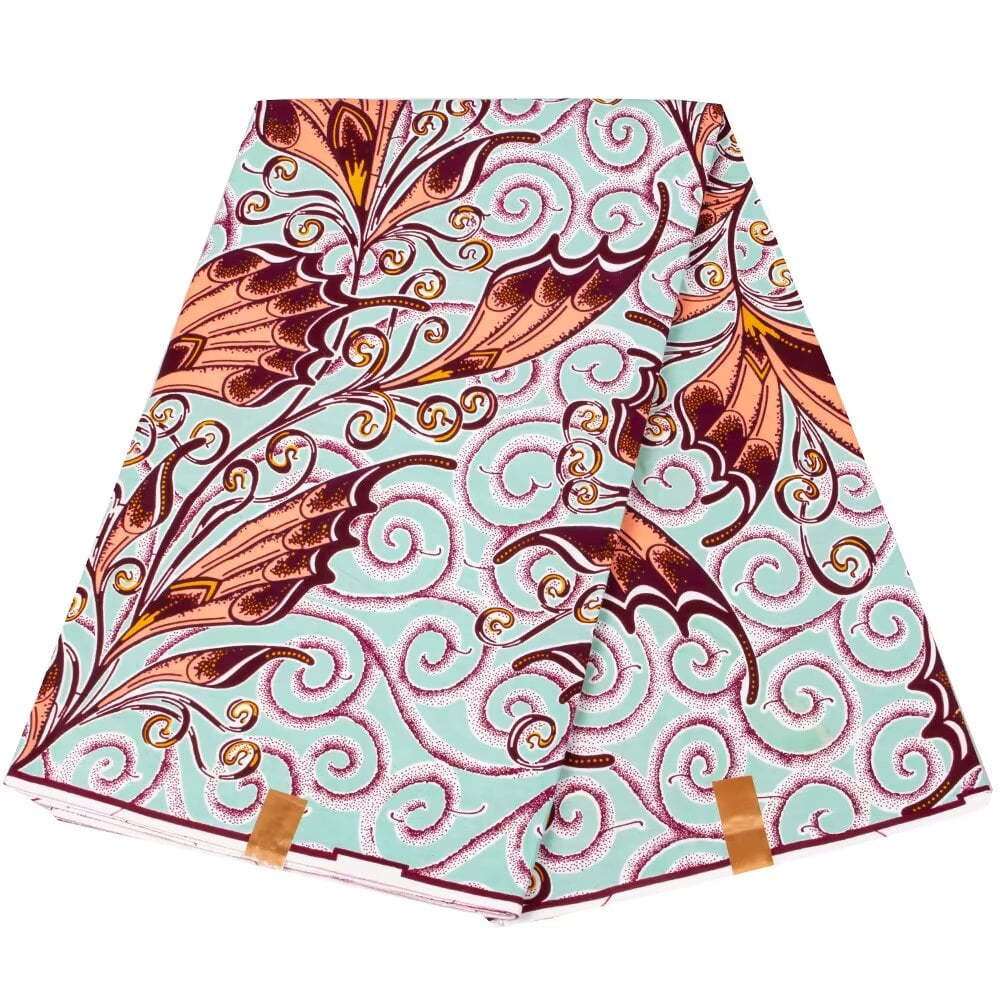The image depicts a piece of folded fabric set against a plain white background, centered in the photo without any borders. The cloth appears to be split into two sections, folding over itself with each edge seemingly taped or banded with brown strips resembling band-aids. The fabric's primary color is light teal or blue, adorned with intricate patterns that include white and brown swirls, as well as leaves that transition from brown to a dark red or orange hue at the tips. Additionally, threads of various colors, including light brown, dark brown, rose gold, dark purple, and gold, interlace the fabric, adding to its rich, multicolored texture. A subtle red line can be seen towards the bottom edge before the white part begins. Despite the visually busy texture, the fabric remains the clear focal point of the image.